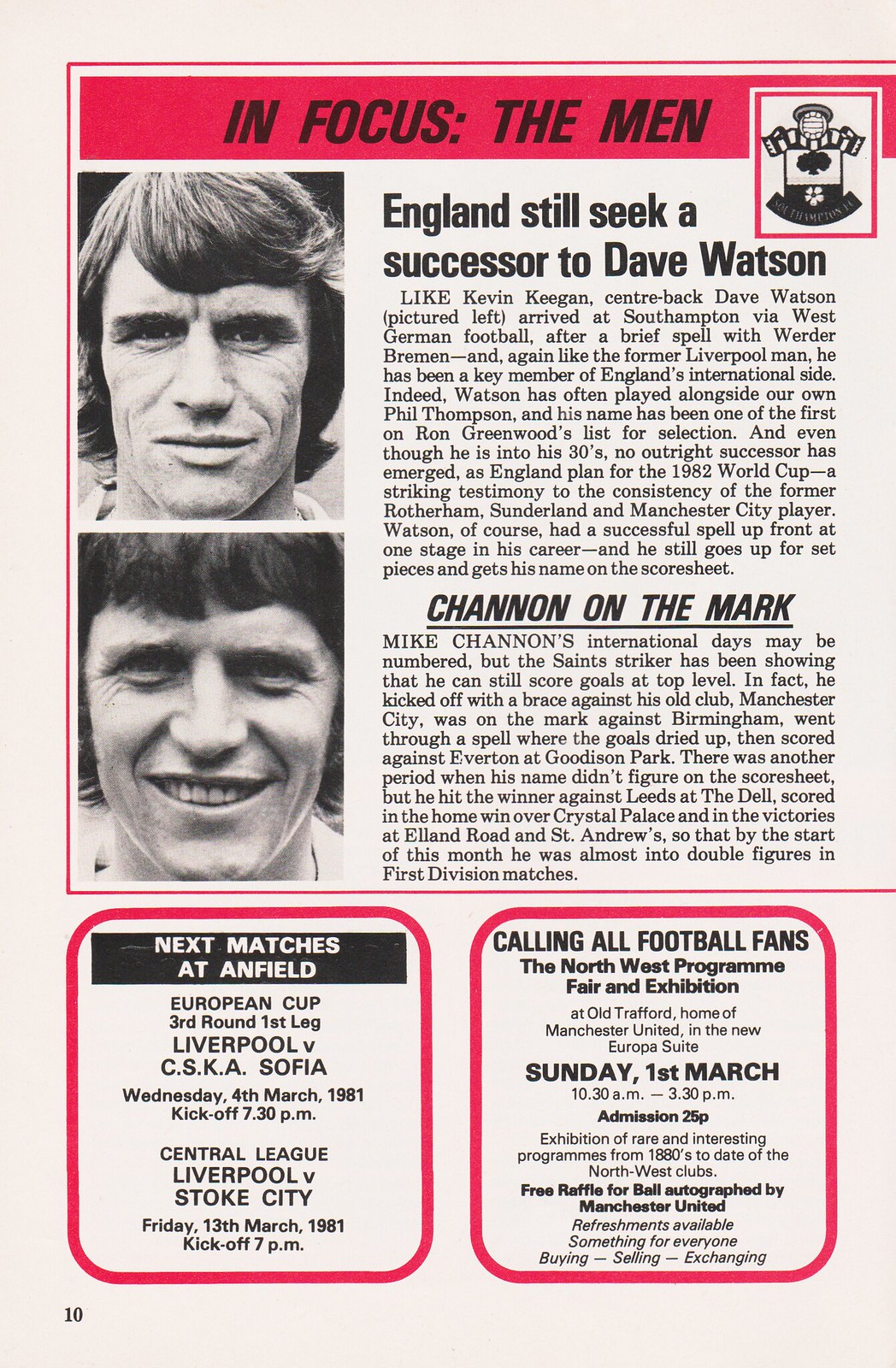The scanned image showcases a detailed, red-accented page from a football program, featuring two stacked pictures of men on the left-hand side. The top section titled "In Focus: The Men" discusses England's search for a successor to center-back Dave Watson. It notes Watson's journey through clubs like Rotherham, Sunderland, and Manchester City and his tenure in West German football with Werder Bremen before joining Southampton. Despite being in his 30s, Watson remains a vital part of England's international side, often paired with Phil Thompson, and is a consistent choice for Ron Greenwood's selection in the lead-up to the 1982 World Cup. Watson, who also had a successful stint playing up front, continues to score from set pieces.

The second section, "Shannon On the Mark," details the exploits of Saints striker Mike Shannon. Shannon, who began the season scoring a brace against his former club Manchester City, also netted goals against Birmingham, Everton at Goodison Park, Leeds at the Dell, Crystal Palace at home, and during away victories at Elland Road and St. Andrew's. Despite occasional dry spells, he was nearing double figures in first division matches by the start of the month.

The bottom left corner lists upcoming matches: the European Cup third round first leg between Liverpool and CSKA Sofia on Wednesday, 4th March 1981, and a Central League game between Liverpool and Stoke City on Friday, 13th March 1981. The right side advertises the "Calling All Football Fans" Northwest Program Fair and Exhibition at Old Trafford, home of Manchester United, on Sunday, 1st March from 10:30 a.m. to 3:30 p.m., featuring rare and interesting programs, a free raffle, and refreshments. The page number "10" is displayed in the bottom left corner.